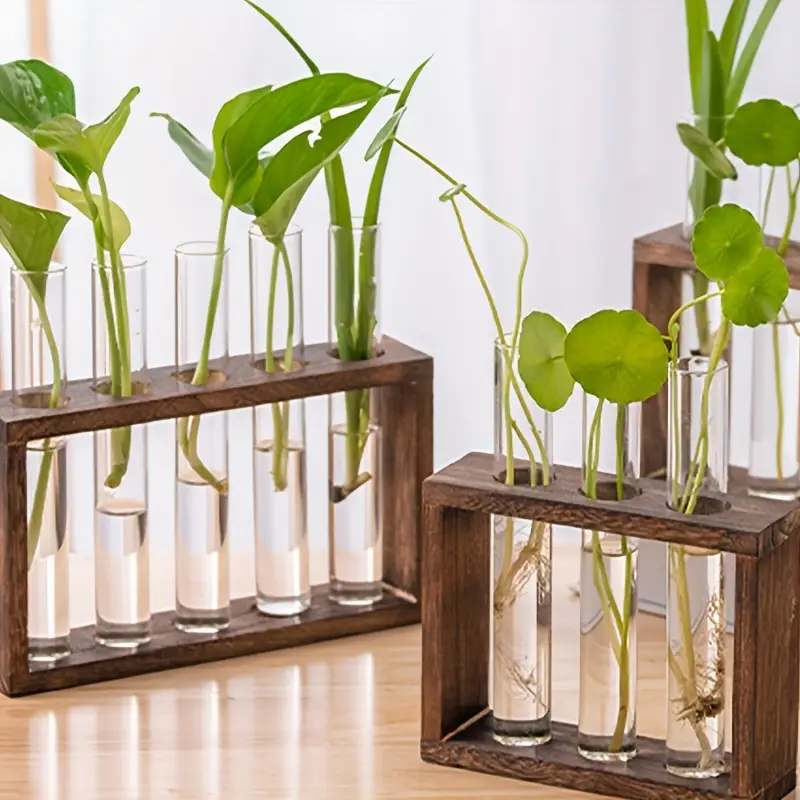The image depicts an elegant setup of various plants being cultivated in clear liquid-filled test tubes. These test tubes, which are either transparent or slightly translucent, are neatly organized within three dark-stained wooden racks, meticulously positioned on a light brown table. Each test tube contains a plant with roots submerged in the clear liquid and green leaves of diverse shapes emerging above: some narrow and elongated, others round or triangular. The table stands against a pristine white wall, which accentuates a stripe pattern faintly visible on the left side, adding a subtle touch to the background. The number of test tubes varies across the racks—one rack holds three test tubes, another five, while the third rack in the background has an undetermined number. The overall composition highlights the growth and variety of the plants within a minimalist and well-structured environment.